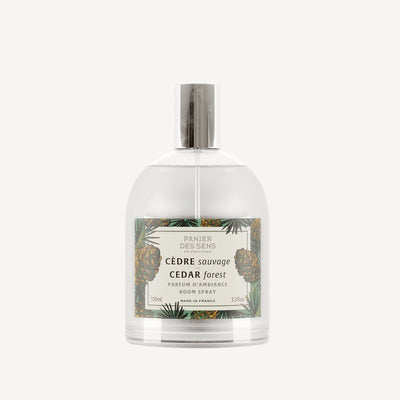The image showcases a slightly blurry, low-resolution product photo of a room spray bottle against a light grey, nearly white background. The bottle is made of clear glass, domed at the top, and filled with a clear liquid. It features a long, cylindrical cap that has a chrome or silver finish. Attached to the cap is a clear plastic tube that extends into the liquid, indicating it is a spray bottle.

The front label of the bottle is square, bordered with illustrations of leaves and pine cones. The center of the label is white, displaying the text "Panir Descense" at the top, followed by "Cedre Sauvage," which translates to "Cedar Forest" in English. Below this, in smaller French writing, is "Parfum D'Ambiance," with the English translation "Room Spray" directly underneath. The bottom left corner of the label appears to state "100 milliliters," although it is challenging to read due to the pixelation of the image.